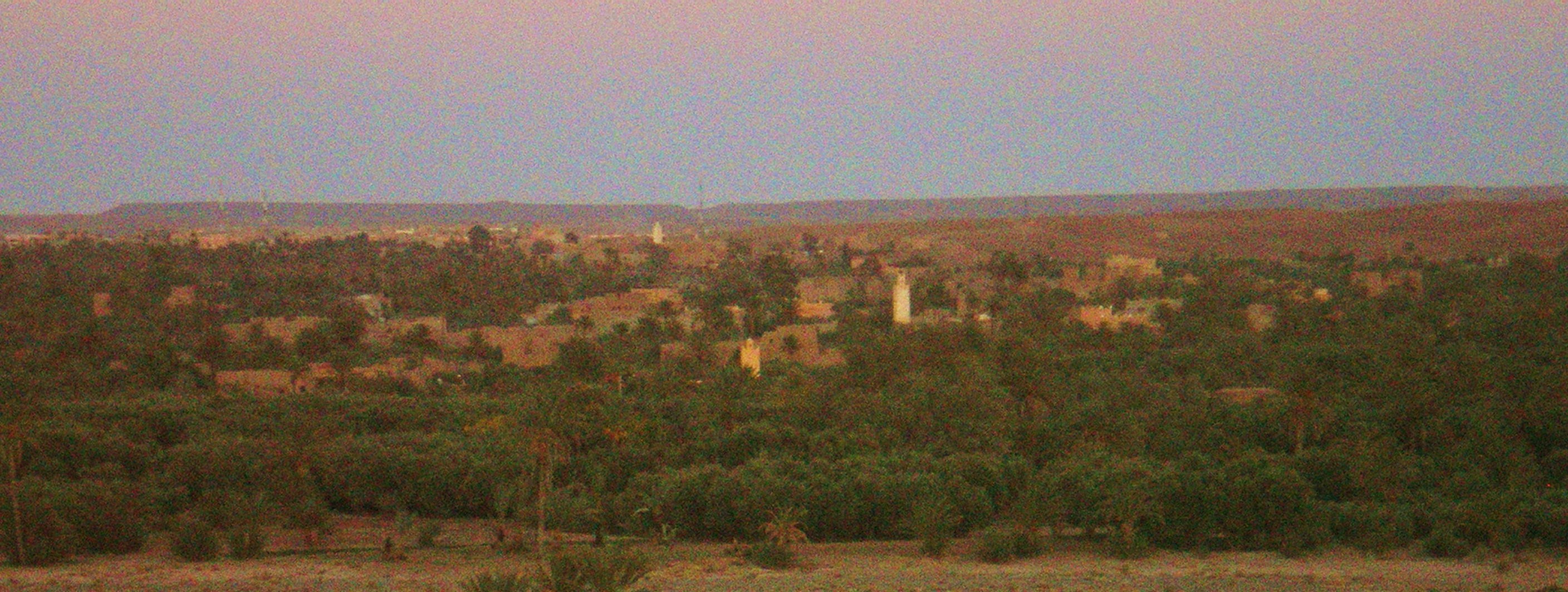This photograph, taken from an elevated vantage point in landscape orientation, depicts a distant outdoor scene of a city surrounded by expansive natural areas. The majority of the ground is densely covered with green trees and various plants, interspersed with patches of brown soil or dry grass. Scattered throughout the greenery are sparse man-made building structures, visible but not plentiful. The clear blue sky above the city shows no clouds and has a subtle grainy quality, with a faint reddish tint suggesting it may be nearing the end of the day. The overall graininess of the entire image enhances the scenic, far-off perspective.